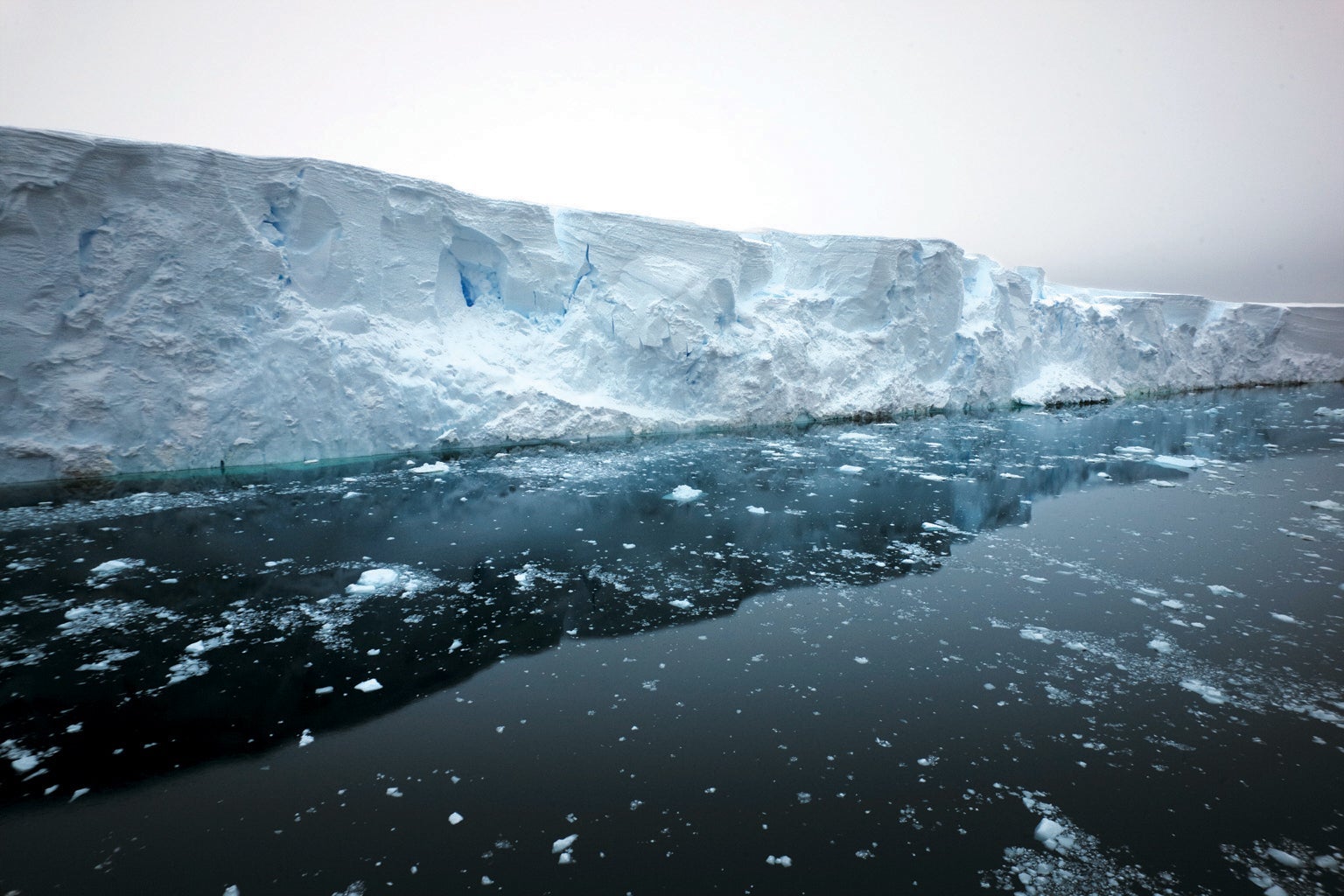This photograph captures a striking outdoor winter scene dominated by a massive, 20-30 feet tall ice wall on the left that appears to rise from frozen, dark blue water. The foreground features a still, icy water surface dotted with blobs and streaks of powdered ice. Stretching horizontally across the image, the ice wall tapers downward and merges seamlessly into the water, which mirrors its formidable presence. The background showcases an overcast sky, painted in a gradient of white and gray, adding to the frosty ambiance. The subtle sun shining through the clouds lends a faint reflection of the ice wall on the dark, almost black, water below, enhancing the serene and frozen landscape.